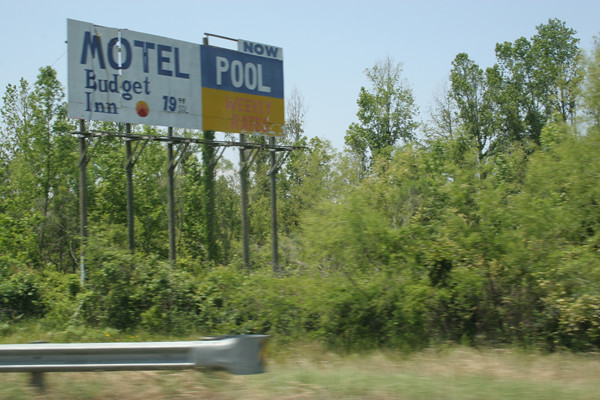A scenic roadside view features a light-colored sky above a lush landscape filled with green trees and bushes. The scene includes a metal side rail along the road, leading the eye to a prominent sign propped up by five sturdy poles. The sign advertises the "Motel Budget Inn" in bold blue letters on a white background, accompanied by a small, vibrant sun icon in yellow and orange. The rate displayed on the sign reads "$79.99." Above the main sign, a smaller white square sign declares "NOW" in blue letters, while below, a blue sign announces "POOL" in white letters. The very bottom of the larger sign showcases an additional yellow section, completing the informative roadside display.